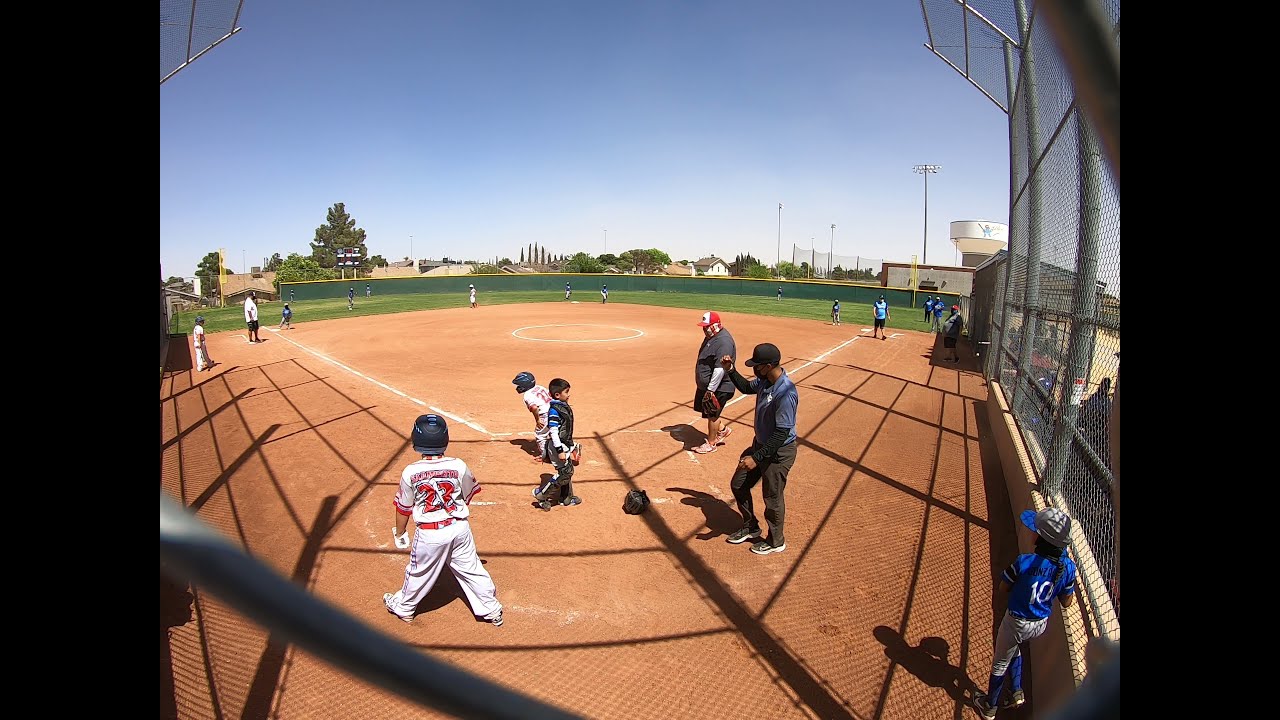This image captures a lively Little League baseball game in progress, viewed from directly behind the catcher’s position. The scene is filled with young players in two distinct team uniforms. One team sports blue jerseys with white numbers, while the other wears white jerseys with red letters and accents, highlighted by a player wearing number 23, who has his back to the camera and dons a black helmet and batting glove. Opposite him at the bottom right is another player, number 10, dressed in blue, also facing away from the camera.

In the center of the image, the catcher, clad in blue protective gear, squats behind the batter in white. Visible to the right of the catcher is the umpire, one hand raised and the other lowered, adding a dynamic touch as he appears almost in mid-dance. 

Two adults, presumably coaches, stand on the field near the batter's box. One man, positioned at first base, wears a blue short-sleeved shirt over a long-sleeved black shirt, paired with black pants and a black cap. The other man, stationed at third base, is much larger and outfitted in a black shirt over a long-sleeved white undershirt, black shorts, and a red and white baseball cap. He also holds a baseball glove, suggesting he might be actively participating in practice or guiding the players.

The field is well-marked with white chalk lines delineating the infield and outfield, as well as the coach's boxes near first and third bases. In the background, a clear blue sky stretches above, with a few trees and buildings visible beyond the chain-link fence framing the right side of the image. This well-organized yet spirited scene encapsulates the essence of youth baseball, combining teamwork, coaching, and the joy of the game.